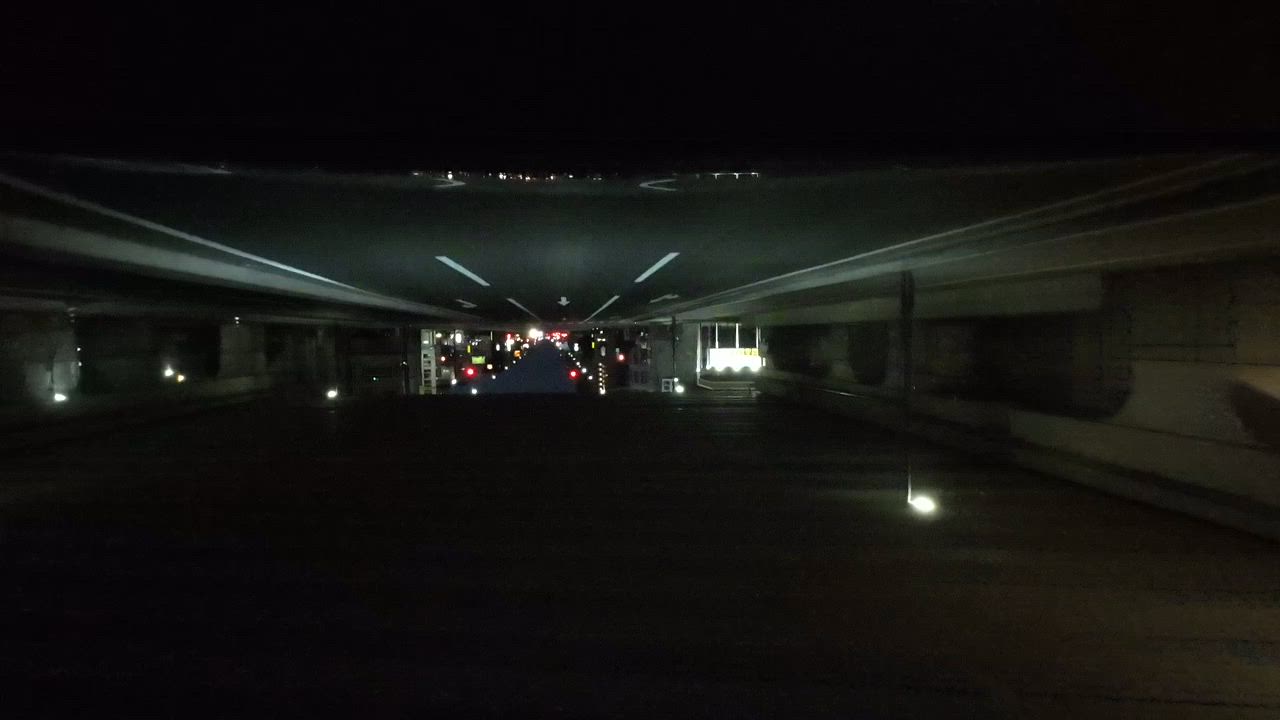The image presents an inverted perspective of a dimly lit scene, creating an illusion that challenges the typical orientation of urban landscapes. The upper portion of the image, which seems to be upside down, depicts a road with clearly visible white lane markings and directional arrows pointing straight ahead. These road elements are juxtaposed against tall buildings illuminated by numerous lights in the distance. The lower part of the image resembles the dark, almost black or dark gray, interior of a garage or tunnel floor. This intriguing play on perspective blurs the lines between the typical and the surreal, engendering a sense of disorientation and curiosity.